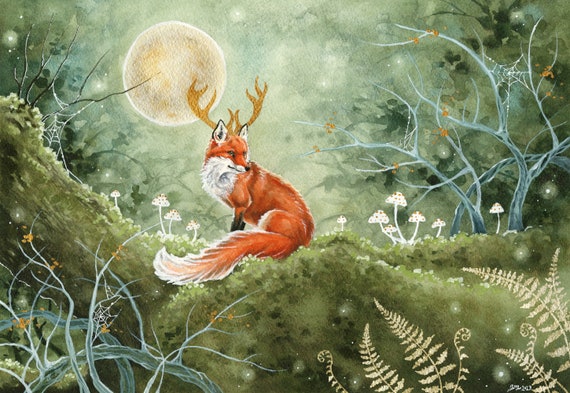In this artistically crafted image, the central focus is an intricately designed fox with distinctive antlers resembling those of a reindeer. The fox, depicted in a side view with its face turned forward, showcases a striking orange fur with white accents on its tail, chest, chin, and the insides of its ears. Positioned in the middle of the composition, it sits upon a green terrain that could be moss-covered. Above the fox, in the top left corner, a luminous white moon rises high, casting an ethereal glow across the scene.

Surrounding the fox, the artistic environment displays a blend of natural elements. The lower part of the image features white ferns and greenish-beige textures, possibly representing hills or mossy ground. Mushrooms in a similar white hue sprout on either side of the fox, contributing to the enchanted forest aesthetic. The borders of the image are adorned with thorny bushes and various gray and white flora, creating a frame that encloses the mystical scene. The sky in the background has a greenish-white tint, further enhancing the moonlit ambiance of this enchanting forest landscape.